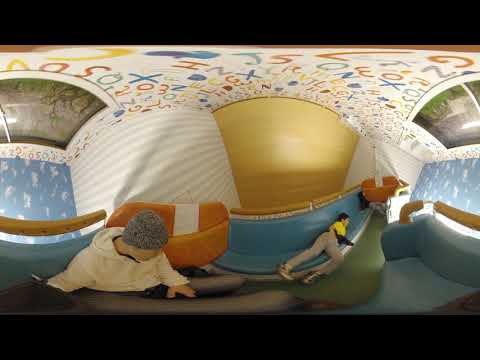The image presents a surreal, panoramic view of an indoor room where the combined curves of the camera lens create a wonky, fisheye effect. On the left side of the frame, a person is seated on a black sofa, dressed in a white hoodie jacket and a black, fur-styled beanie. He is looking to the right. An orange-colored couch with a white square in the center is visible behind him. To his right, another person lies on an elongated blue couch, resting on his left side, which appears as the right to the viewer. This individual wears a yellow shirt with black sleeves, tan pants, and matching shoes, and looks to the right. The room features light blue and beige striped walls, embellished with white decorations. The ceiling is white, adorned with an array of primary-colored numbers and alphabet letters, reminiscent of a playful children's room decor.